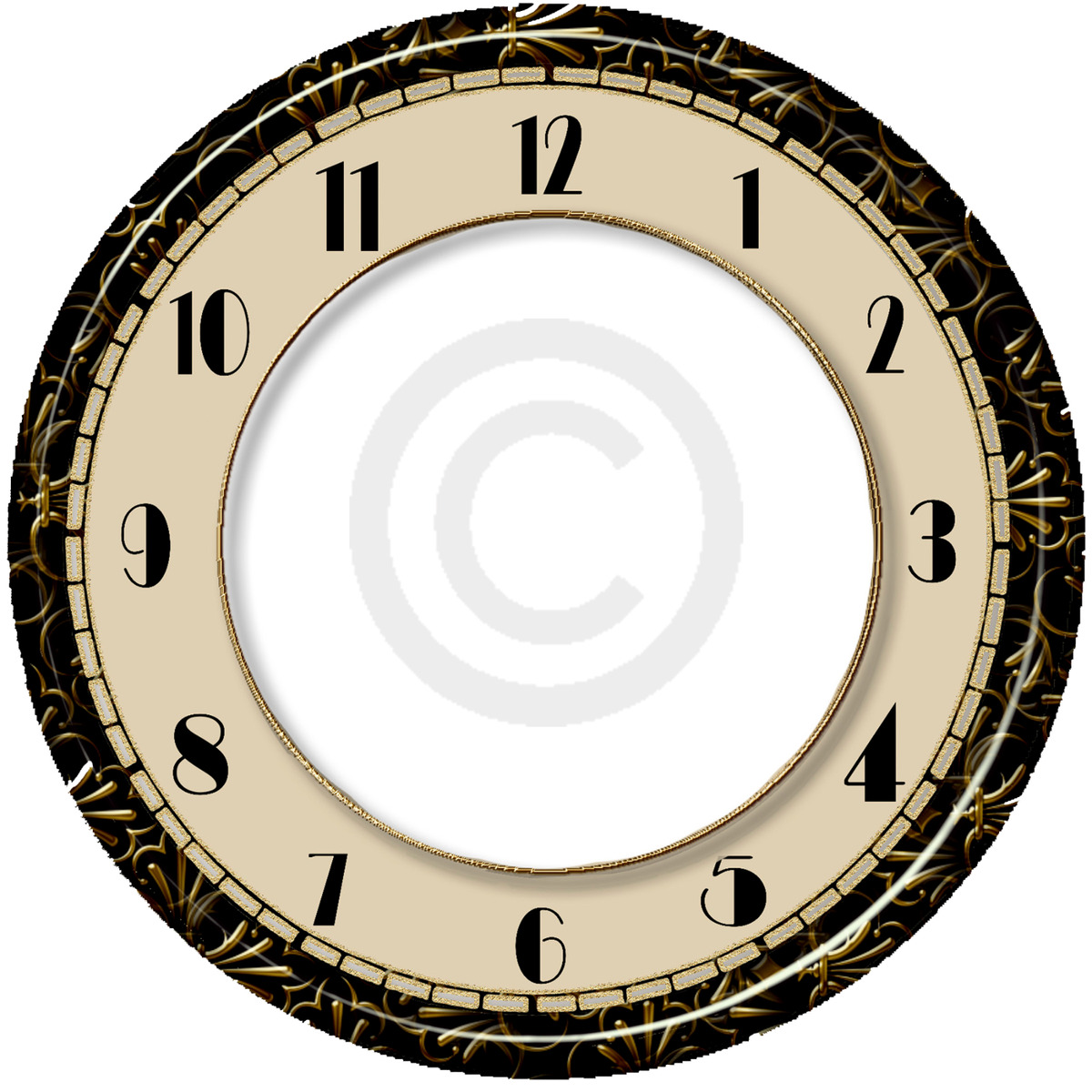The image showcases a circular clock floating against a white background, devoid of a defined border or frame. The exterior edge of the clock features a black border embellished with intricate gold design elements. Inside this, there is a thin, cream-colored border composed of small bars or rectangles interspersed with black lines. Following this, a much wider cream circle displays black, stylized numerals from 1 to 12 arranged in their conventional positions. Encircling this numbered section, there is a delicate gold border, leading to a stark white inner circle at the clock's center. Within this white center, a faint gray circle houses a gray 'C'. Notably, the clock lacks any hour, minute, or second hands, emphasizing its ornamental nature. The rim of the clock, which appears to be made of plastic, is adorned with gold patterns resembling partial flower petals, enhancing its decorative appeal. The overall composition gives the impression of a computer-generated image rather than a traditional photograph.